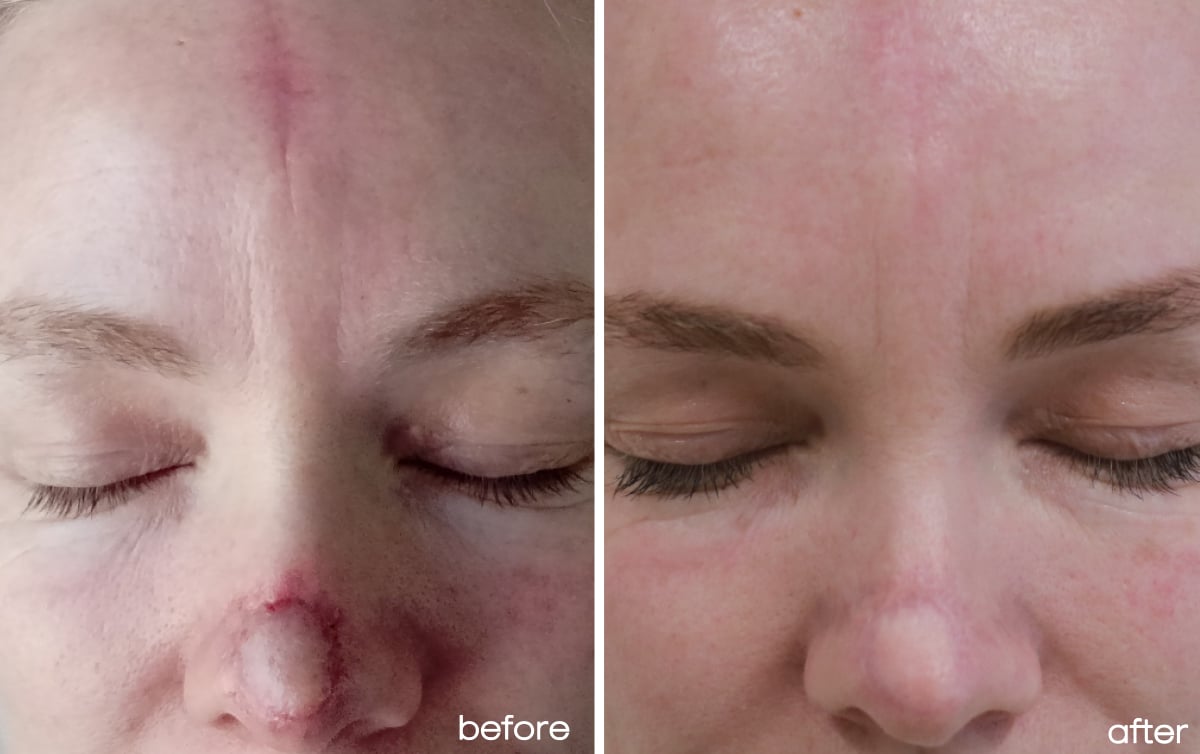The image features a close-up of a Caucasian woman's face, divided into two side-by-side photographs labeled "before" on the left and "after" on the right. The focus is solely on her face, displaying her closed eyes, brown eyebrows, eyelashes, eyelids, and nose. The "before" photo reveals significant facial blemishes and severe redness, particularly highlighting a visibly distressing condition on the tip of her nose, consistent with the aftermath of a surgery such as Mohs surgery. The "after" photo shows dramatic, positive changes—her skin appears much clearer overall, the red marks on her forehead are practically gone, and her nose, which previously seemed severely injured, shows remarkable healing with only a slight scar remaining. The images together seem to serve as an advertisement for a skin treatment or surgical procedure that has effectively improved her condition.